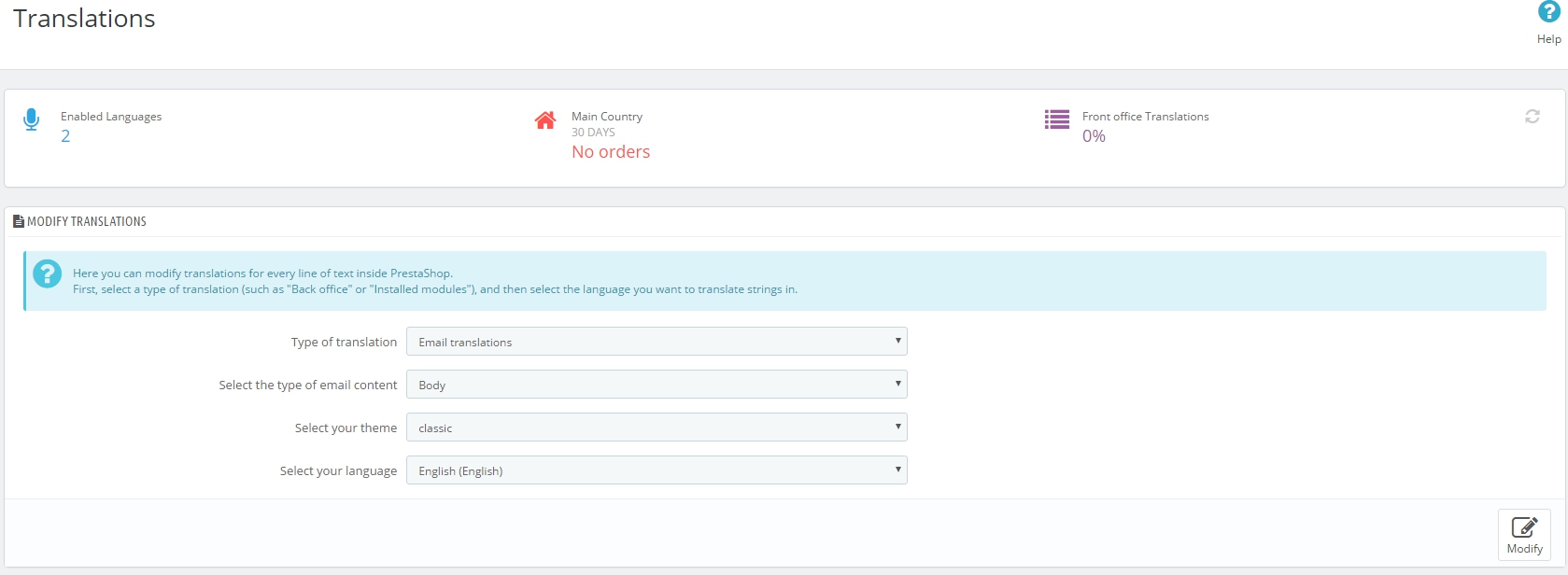This image depicts a screenshot from a computer interface related to translation management, possibly within a PrestaShop environment. The top section prominently displays a heading titled "Enabled Languages," flanked by a blue microphone icon. Directly to the right, the section pertinent to "Main Country" reveals a time frame of "30 days" and indicates "No orders." Next to this area, there's a red house icon. Toward the extreme right of the interface, the header "Front Office Translations" can be seen, accompanied by two decorative purple lines and squares, and showing a progress indicator of "0%."

Below this primary area, there's a section labeled "Modify Translations." Within a teal-colored box, it provides instructions: "Here you can modify translations for every line of text inside PrestaShop. First, select a type of translation such as back office or installed modules, and then select the language you want to translate strings in."

Further down, the interface features four dropdown menus contained within rectangular boxes:

1. The first dropdown menu includes the prompt "Type of Translation" with "Email Translations" selected.
2. The second menu asks to "Select the Type of Email Content," with "Body" chosen.
3. The third box prompts to "Select Your Theme," displaying "Classic."
4. The final dropdown menu allows users to "Select Your Language," with "English" selected.

This detailed display clearly organizes various translation management settings into an intuitive and navigable format.